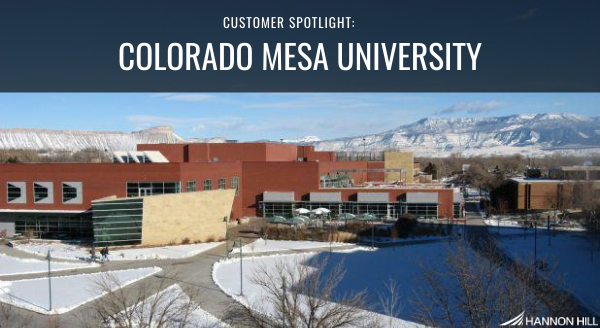The image showcases Colorado Mesa University during winter, prominently featuring a red brick building with lighter wood accents and ten windows outlined in gray, set against a snowy backdrop. The scene is framed by barren trees and light poles dotting the cleared walkways that crisscross the snow-covered grassy areas. At the top of the image, white text reads "Customer Spotlight Colorado Mesa University," highlighting the institution. The background is dominated by majestic mountains capped with snow under a blue sky with patches of gray clouds. The bottom right corner of the image bears the Hannon Hill logo, adding a professional touch to the serene, wintry landscape.